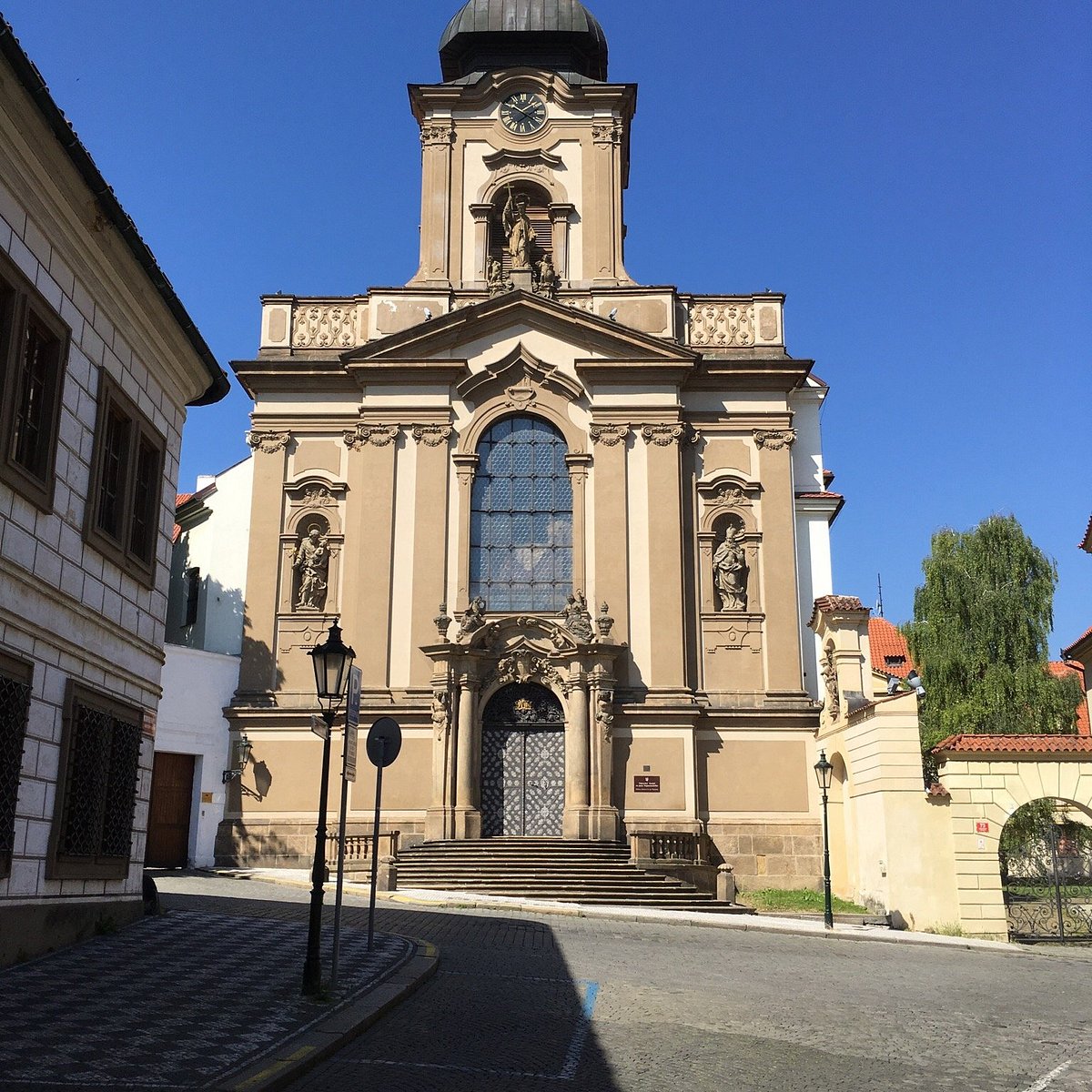The photograph captures a very large and old church building, positioned prominently at the forefront of a cobblestone street, indicative of an old town, likely situated in Northeast America or Europe. The church, standing at the height of a six or seven-story building, features a striking architectural blend with a pointed roof and a dome-like top. The façade is primarily beige or brown, embellished with intricate statues and sculptures of religious figures above the main entrance.

A grand staircase, which varies in the number of steps due to the building's position on a tilted slope, ascends to a pair of black and gray swinging doors adorned with a grid pattern. Above these doors, there is an arch with more statues and elaborate designs, topped by a tall, multi-paneled window that ends in an additional arch. Crowning the structure, a clock with a black face and gold letters is installed, slightly above a brown statue.

In the background, the sky is a perfect blue, underscoring the bright, sunny day without a trace of clouds. To the right of the church, a building with white walls and brown-framed windows can be seen, accompanied by a black streetlight and a partially obscured traffic sign with a red dot. On the far right side stands a lush green tree, its dark leaves adding a natural contrast to the urban landscape. The cobblestone street is fringed by a pedestrian walkway made up of gray and dark gray checkered stone with a small curb, adding to the old-world charm of the scene.